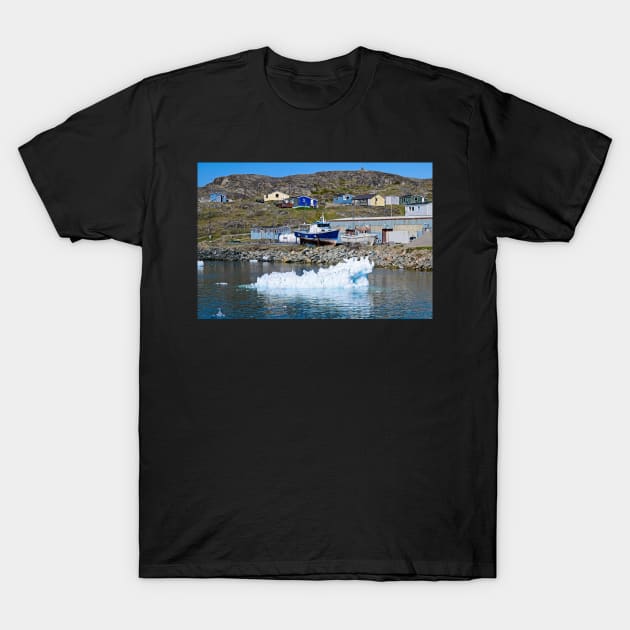This black, short-sleeve t-shirt features a vibrant photograph on the front, capturing a serene ocean shoreline scene that evokes the rugged beauty of Newfoundland. The image displays a rocky shore with several colorful houses prominently perched on a hillside—painted in shades of yellow, blue, teal, and gray. The shoreline includes small buildings and a blue boat that has been pulled onto the land.

In the foreground, the deep blue water showcases a distinct white iceberg, standing out against the calm expanse of the sea. The horizon reveals smaller boats amidst a backdrop of rolling hills, which are dotted with brown, green, and occasional blue hues, likely from wildflowers. Above this picturesque landscape, a clear blue sky stretches out, completing the tranquil and picturesque coastal scene depicted on the t-shirt.